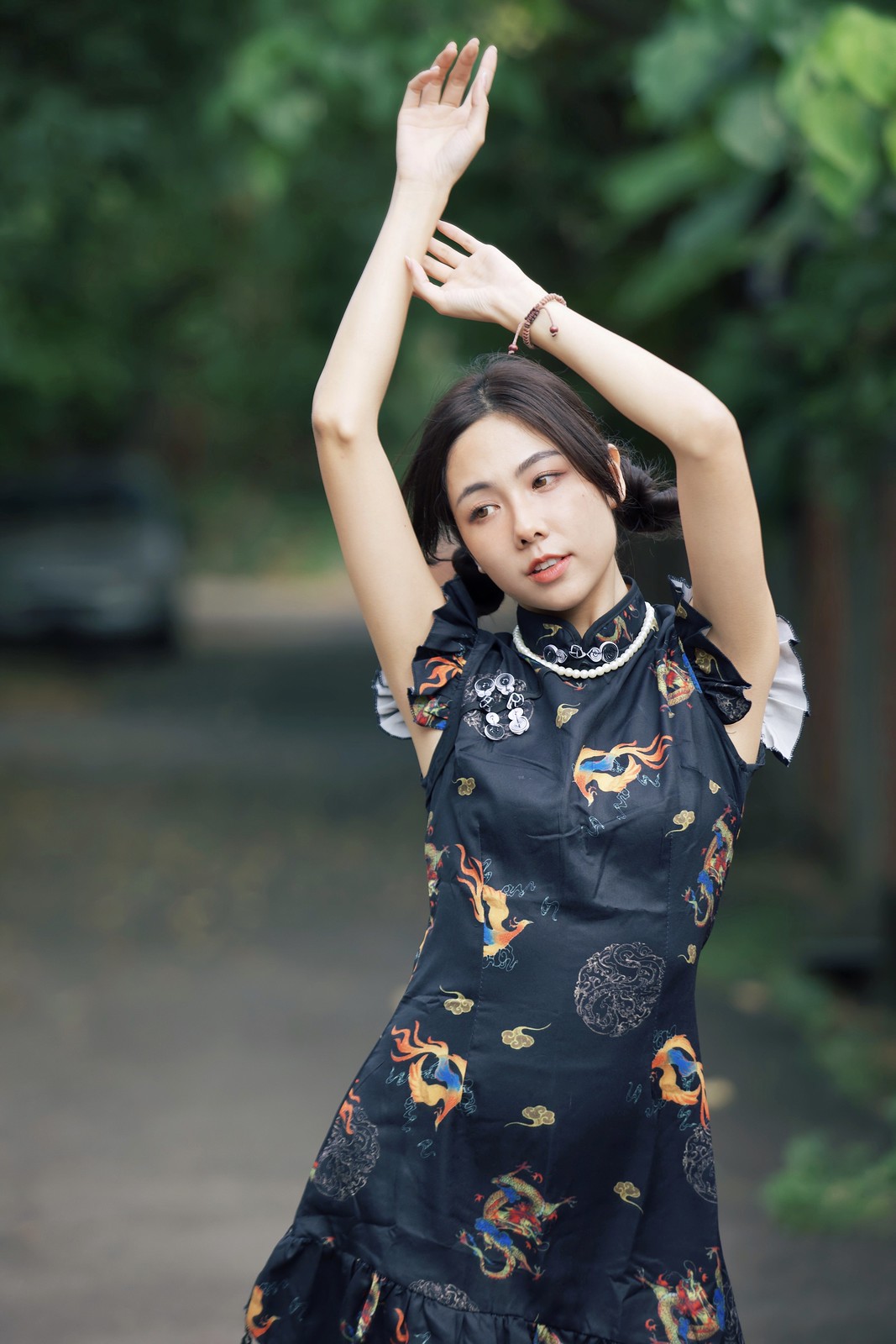This is a professionally taken photograph of a young Asian woman, possibly in her teens or twenties, standing outdoors on a driveway lined with lush green trees. She is wearing a striking, mostly sleeveless black dress adorned with intricate designs resembling Chinese dragons and colorful patterns in shades of orange and blue. The dress has subtle white accents on its sleeves, adding to its elegance. She accessorizes with a pearl necklace draped around her neck and dress, and a bracelet on her left wrist. Her black hair is pinned back slightly but falls down around the sides of her face. In a graceful pose, she raises both hands above her head, with her right hand higher than her left, which gently grasps her right wrist. A blurred car is visible in the background to the left, emphasizing the focus on her. The photograph, taken in daylight, is vertically oriented and highlights her poised demeanor against the serene, tree-lined backdrop.